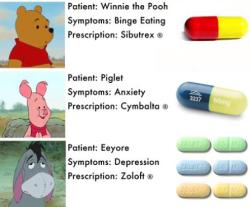On a white background, this image humorously combines medical elements with beloved characters from Winnie the Pooh. On the left side, there are three small thumbnail images of the characters. The first one is Winnie the Pooh, a little bear wearing a red short-sleeved shirt. The second character is Piglet, a pink piglet wearing a pink bow tie. The third character is Eeyore, a sad-looking gray donkey with a tuft of black hair, light gray nose and mouth area, and drooping ears with visible pink insides.

To the right of the characters, there are various pills displayed. These include one red and yellow capsule, one blue and white capsule, two green pills or tablets, two blue pills or tablets, and two yellowish-tan pills or tablets, each with scoring marks for splitting.

In the middle of the image, black text provides mock medical information for each character. It reads: "Patient: Winnie the Pooh, Symptoms: Binge Eating, Prescription: Sibutrex™," accompanied by the red and yellow pill. Next, "Patient: Piglet, Symptoms: Anxiety, Prescription: Cymbalta®," matched with the blue and white pill. Finally, "Patient: Eeyore, Symptoms: Depression, Prescription: Zoloft®," with two of each color tablet (green, blue, and yellowish-tan).